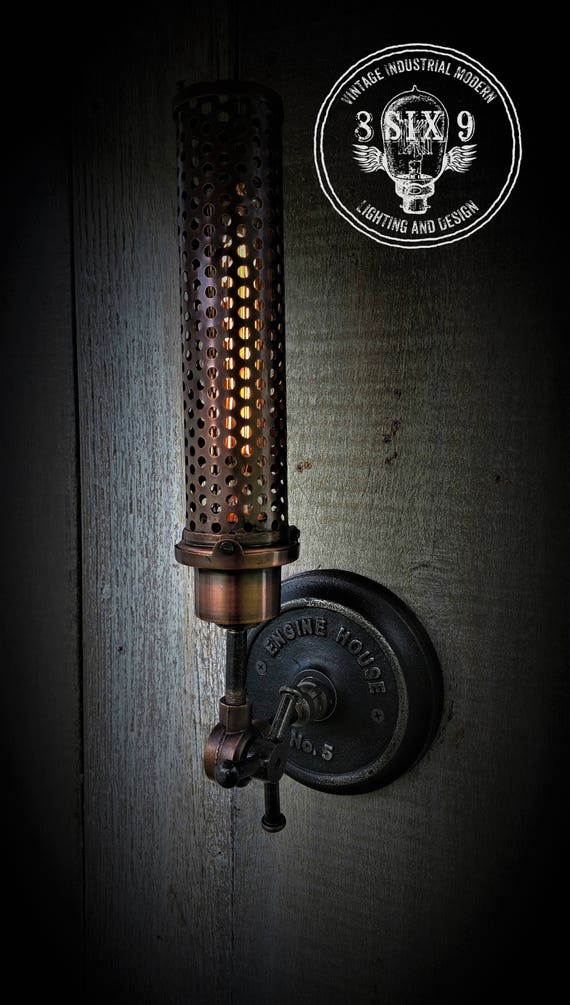This image showcases a unique, antique-style light fixture mounted on the exterior of a wooden structure. The dark, unfinished wood paneling, with hues of gray and green, serves as a rustic backdrop for the fixture. The light is attached to a thick, round metal base painted black, which is engraved with "Engine House Number 5."

The light fixture itself embodies a vintage aesthetic. It features a cylindrical shape with a shiny dark brown, almost bronze, finish accented with hints of brass. Encasing the light is a metal mesh grate of a matching brassy dark brown color, providing a glimpse of the glowing yellow light within.

Prominently displayed in the upper right-hand corner of the image is a white circular emblem. This emblem reads "Vintage Industrial Modern Lighting and Design," encapsulating an old-fashioned light bulb with wings and the number 869 emblazoned above it. This logo suggests that the light fixture is a product of this company, known for its industrial and vintage design elements.